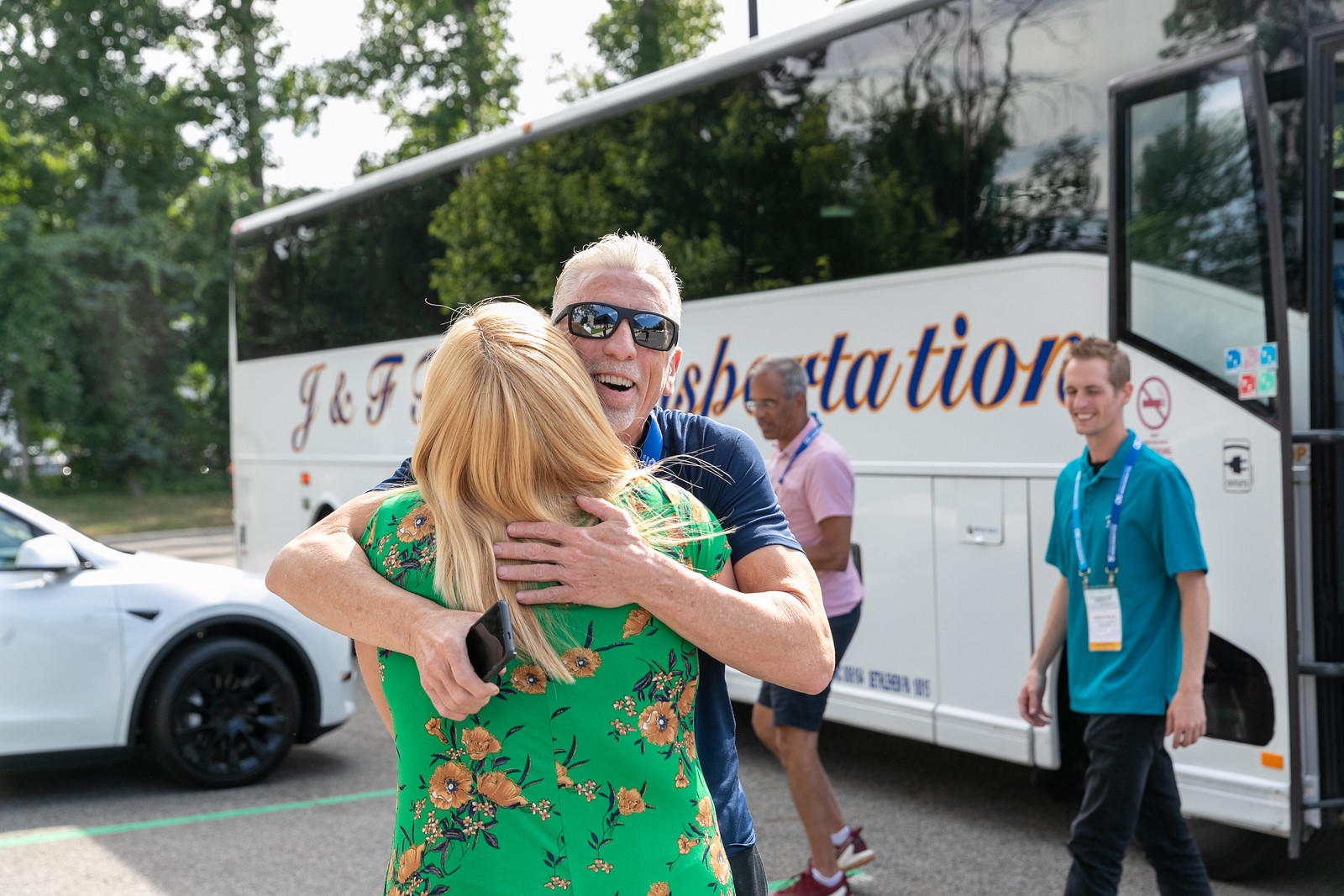In the foreground of this photograph, a heartwarming embrace takes place between a younger blonde woman and an elderly man. The woman, seen from behind, boasts shoulder-length blonde hair and dons a vibrant kelly green dress intricately adorned with gold flowers and green leaves. She hugs the man, who sports white hair and a broad smile. He wears dark, mirrored sunglasses and a short-sleeved dark blue shirt, holding a black cell phone in his right hand. His joy is palpable as he warmly returns the hug.

The setting is a bustling parking lot, immediately in front of a large white bus bearing the inscription "J and F Transportation." Additional figures populate the background: a tanned individual with gray hair in a pink shirt and blue shorts, sporting red sneakers, and another person in a blue polo shirt smiling at the embracing pair. The bus features black mirrored windows reflecting green trees in the background, and the scene is further detailed with a white car with black tires positioned to the left of the embracing couple.